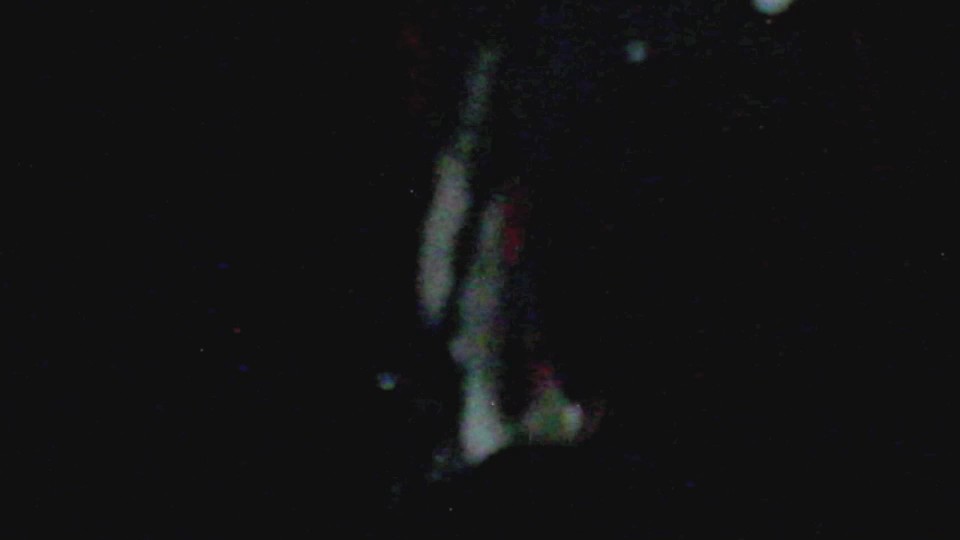In this dark, eerie image dominated by blackness and speckled with various colors, the central focal point is a mysterious, indistinct figure. The figure's shape is reminiscent of an upside-down lily, with a white, dress-like appearance at its base and hints of red hues above it, contributing to an unsettling vibe. There are noticeable white dots, possibly lens flares, hovering above and to the right of the figure. The image is grainy and low in quality, with specks of blue, red, and white scattered throughout the black backdrop, adding to the confusion and distortion. This hazy, ghost-like figure is surrounded by abstract shapes and colors, heightening the overall sense of creepiness and ambiguity within the composition.